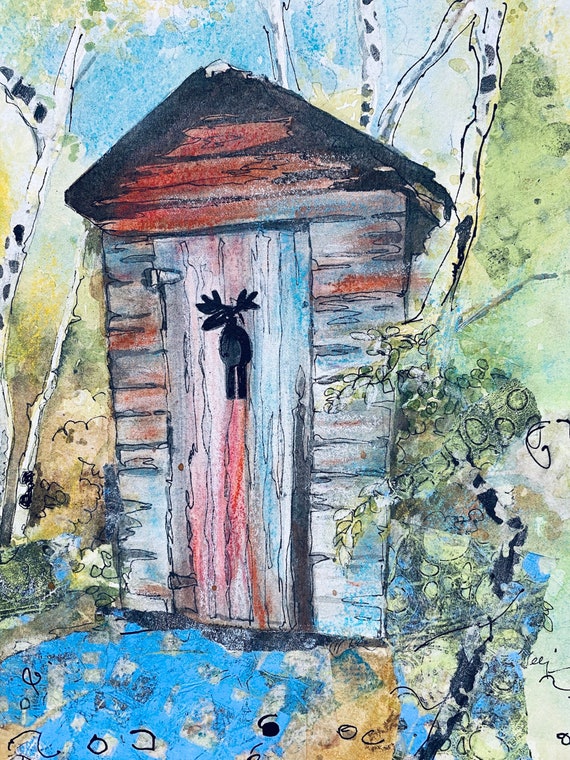This whimsical watercolor illustration depicts a quaint outhouse constructed from various shades of unfinished wood, ranging from browns to hints of red and green. Notably, the outhouse door features a playful cutout in the shape of a moose, complete with antlers, reminiscent of traditional outhouse designs but with a unique twist. Surrounding the outhouse are clusters of white trees, likely aspens or birches, characterized by their distinctive black spots. The ground around the structure is highlighted with blue shading, suggesting a pathway leading to the door. Lush green bushes and foliage encircle the scene, adding bursts of green alongside the trees and in front of the outhouse. The background features a clear blue sky, indicating a bright and sunny day, contributing to the overall whimsical, cartoon-like charm of the painting.